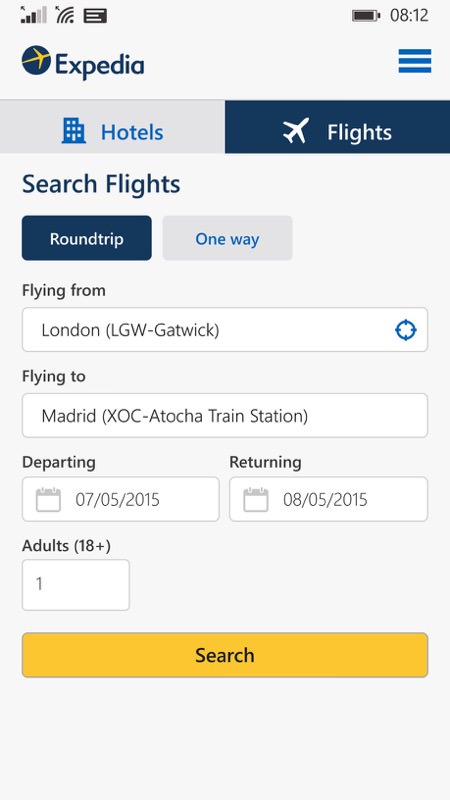The image displays a phone screen showing a webpage from the Expedia website. At the top, the status bar indicates that Wi-Fi is enabled, the battery is nearly full, and the time is 8:12, though it is unclear whether it is AM or PM. The Expedia logo, characterized by a blue circle with a yellow airplane, is prominently featured. A menu button, symbolized by three blue lines, is located near the logo.

Beneath the Expedia header, two options are available: "Hotels" and "Flights." "Hotels" is shown in a gray box with blue text, while "Flights" is highlighted in a blue box with white text. Below these options, a section for searching flights is displayed, with "Round Trip" selected in dark blue with white text, and "One Way" in gray with blue text.

The flight details are filled out as follows: the departure city is London, with Gatwick Airport (LGW), and the destination is Madrid, with Atosha Train Station (XOC). The departure date is listed as July 5, 2015, and the return date as August 5, 2015. The number of adults traveling is set to one, and all this information is presented in black text within white boxes.

At the bottom, there is a prominent yellow search bar with black text, suggesting that clicking it would generate a list of flight options matching the entered criteria.